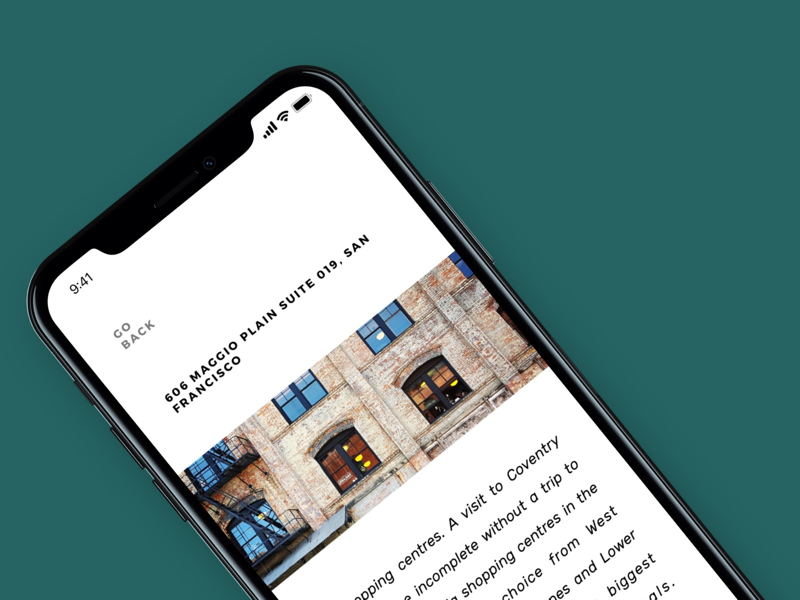The image depicts a smartphone displaying a webpage, likely an advertisement. The webpage provides an address: "606 Maggio Plain Street, 019 San Francisco." Below the address, there is a photograph of a building, possibly the location at the specified address. Accompanying the image is a promotional text that reads: "A visit to the conventory is incomplete without a trip to the San Francisco Shopping Center, the choice of the west." The overall design suggests a marketing campaign aimed at promoting the highlighted location and nearby attractions.